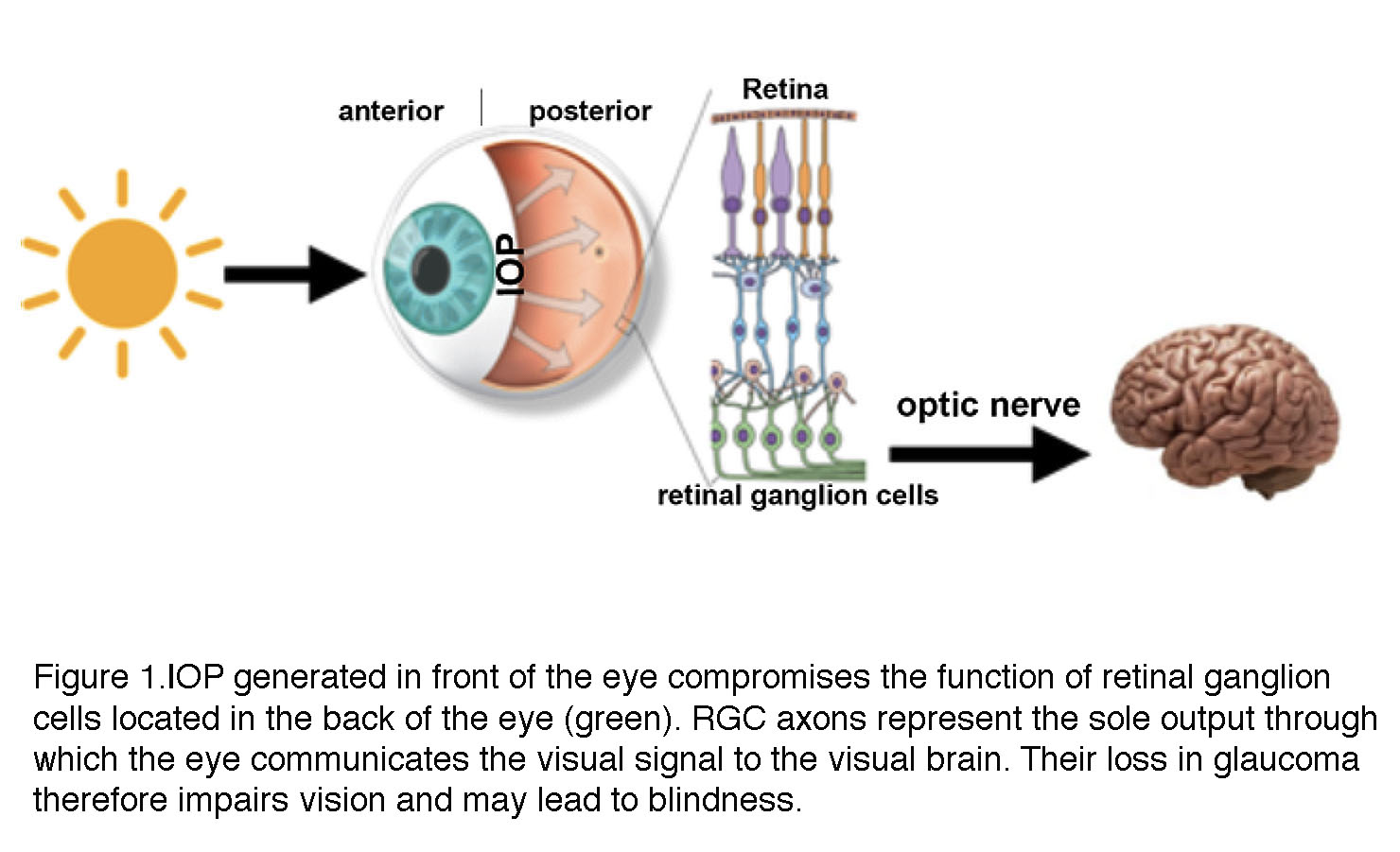The diagram illustrates the process of visual perception from the eye to the brain. On the left, a yellow sun emits rays indicated by a black arrow pointing towards an eyeball. The diagram labels the anterior and posterior sections of the eyeball, including the iris. The rays pass through these parts, reaching the retina at the back of the eye. The retina contains retinal ganglion cells, shown in green, which send signals through the optic nerve, depicted by another black arrow, towards a pink brain on the right. Accompanying this visual representation, there are detailed annotations: "Figure 1 OP generated in front of the eye compromises the function of retinal ganglion cells located in the back of the eye green. RGC axons represent the sole output through which the eye communicates the visual signal to the brain. Their loss in glaucoma impairs vision and may lead to blindness." This conveys the critical role of retinal ganglion cells and the potential vision loss due to glaucoma. The diagram combines bright green, yellow, and purple coloring for emphasis, enhancing the clarity of its educational message.